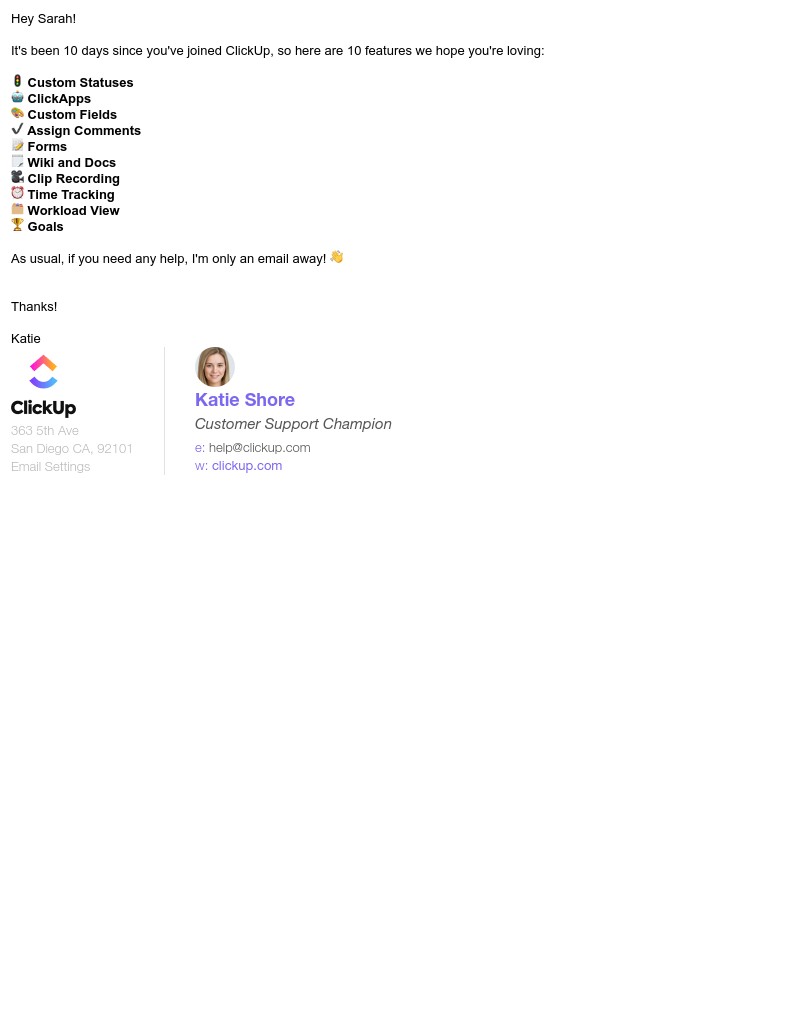This screenshot from a website features a welcoming message on a clean white background. At the top, the text says "Hey Sarah!" in bold black letters. Following this greeting, it informs Sarah that it has been 10 days since she joined ClickUp. The text clarifies that "ClickUp" is a single word with both the 'C' and 'U' capitalized.

The main body of the message lists ten features that the website hopes Sarah is enjoying:
1. Custom Statuses
2. Click Apps
3. Custom Fields
4. Assign Comments
5. Forms
6. Wiki and Docs
7. Clip Recordings
8. Time Tracking
9. Workload View
10. Goals

The message then extends an offer for further assistance: "As usual, if you need any help, I'm only an email away. Thanks, Katie."

At the bottom left of the message, there is a graphic displaying an upward arrow with a smile beneath it, alongside the ClickUp logo. The company's address is also provided. On the right side, the sender's information is displayed, showing "Katie Shore, Customer Support Champion," along with her email (denoted as "E:") and the website (denoted as "W:"). Above this information, there is an image of Katie's face from the neck up.